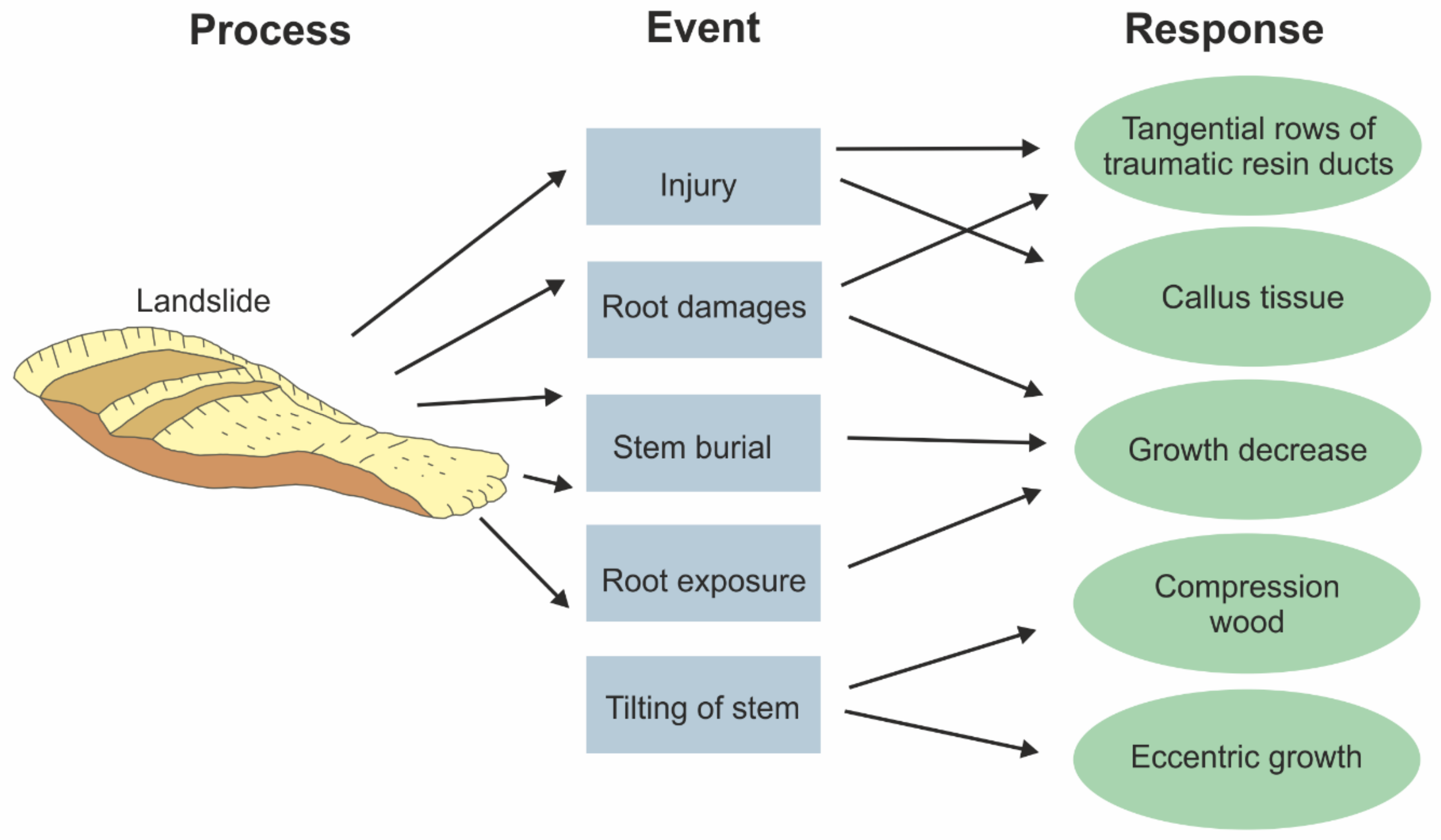The illustration is a detailed depiction of a landslide process and its subsequent effects, resembling a graphic commonly found in a science textbook. On the left side, marked with the heading "Process," there is an image illustrating a landslide. Arrows from this illustration point to the center column labeled "Event," which contains five blue boxes with the following designations: injury, root damages, stem burial, root exposure, and tilting of stem. From each of these boxes, further arrows extend to the right column under the heading "Response," leading to five green oblongs that detail the subsequent responses: tangential rows of traumatic resin ducts, callus tissue, growth decrease, compression wood, and eccentric growth. The diagram effectively traces the sequence from the initial landslide through to various biological and ecological responses.